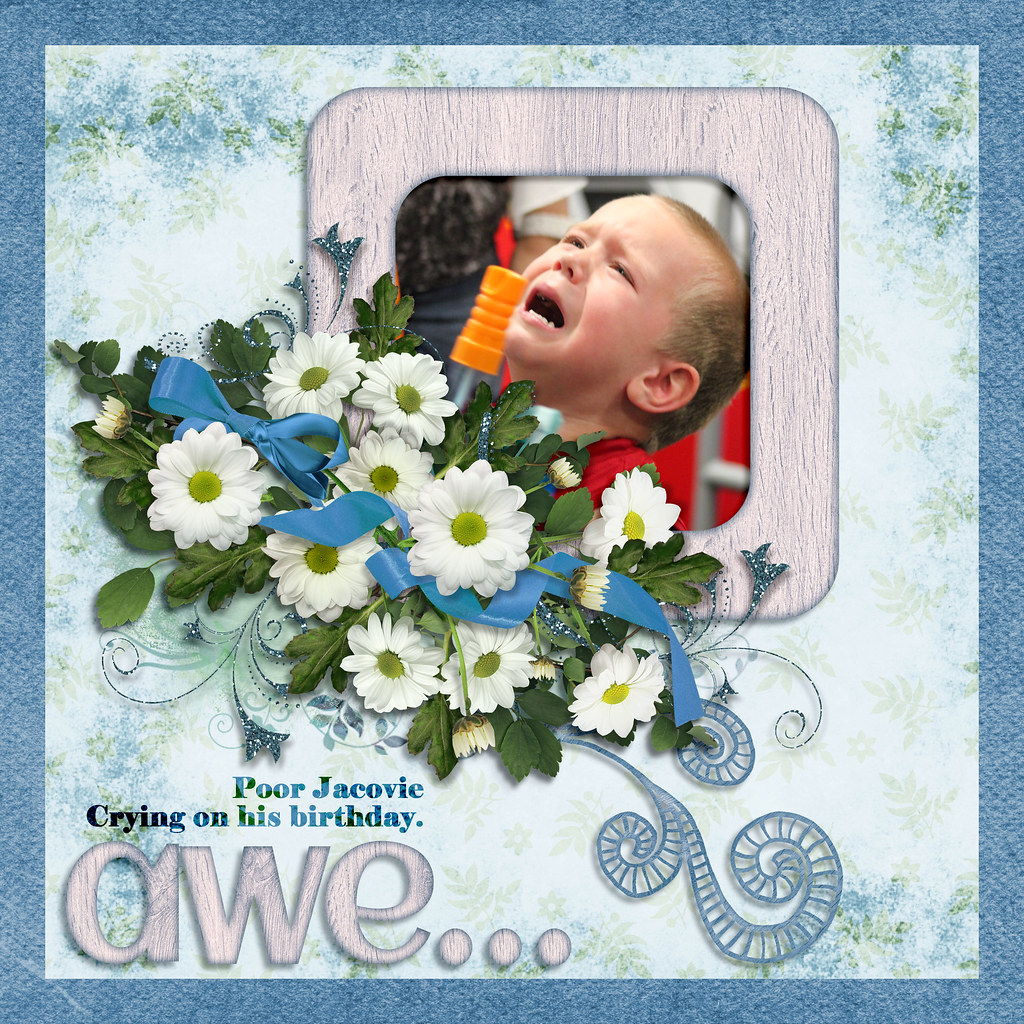The image appears to be a digital or physical greeting card, likely intended for social media or family sharing, featuring a young boy, approximately three or four years old, crying and looking upwards as if in distress. He is depicted within a gray, wooden frame-like border. Below the boy's framed photo is a bouquet of white daisies with green centers, tied together with a blue ribbon, positioned at the bottom left corner of the frame. The background of the image is a textured light blue with shades of blue and green, giving it a calming yet melancholic tone. The border surrounding the image is a solid blue. Text at the bottom left corner reads, "poor Jacobi crying on his birthday," in small blue letters, and directly below it, in large gray letters, it says, "awe..." in an affectionate, drawn-out manner. The boy is wearing a red shirt, adding a striking contrast to the blue and green hues of the background.